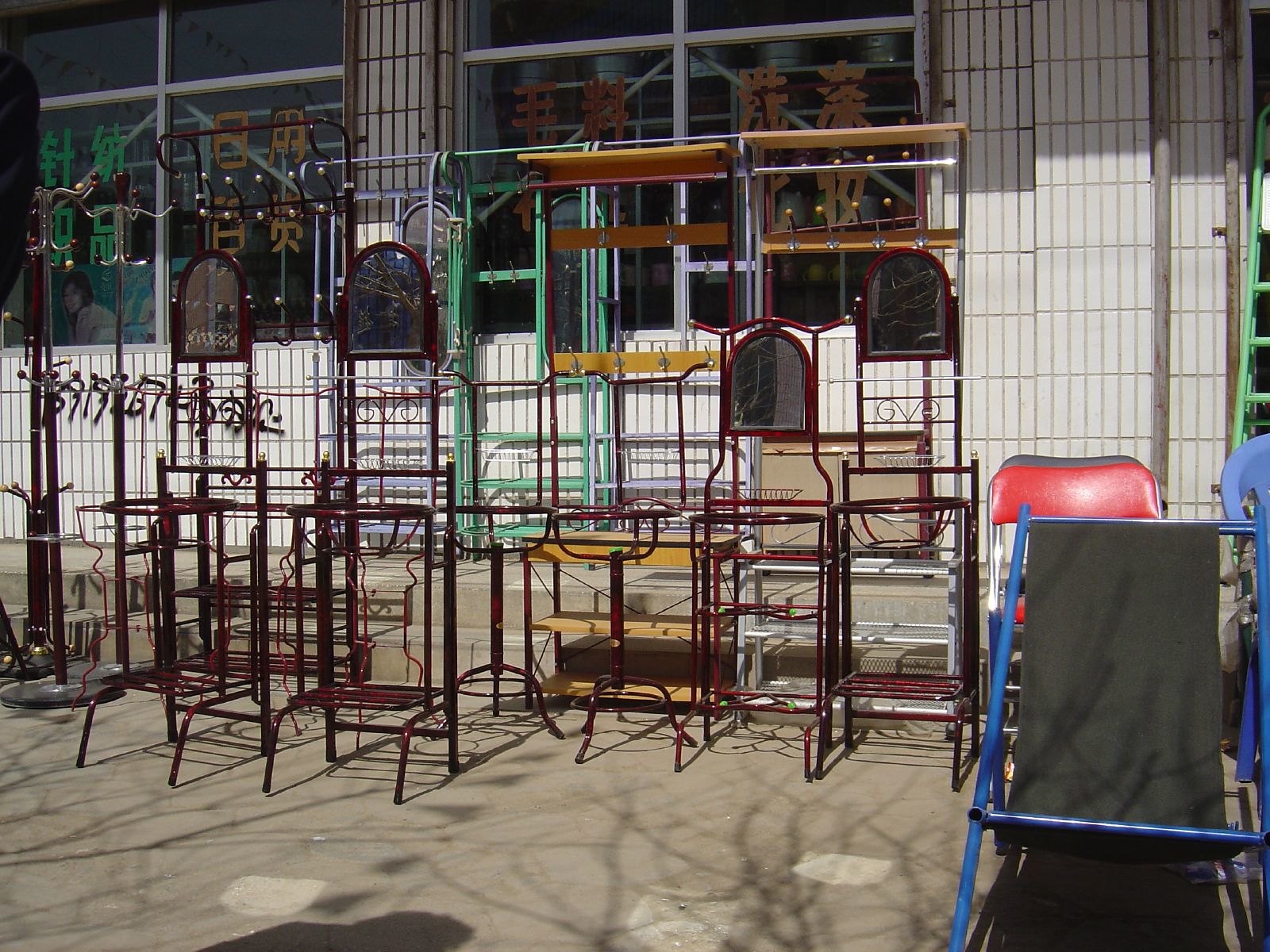The photograph depicts an outdoor market-like setting in front of a building with a metal, white (possibly off-white) facade. The backdrop features large glass windows adorned with text that appears to be in Chinese or Korean characters and an image of a smiling woman, likely part of the store's signage. Spread across a large concrete area in front of the building are various metal shelving units arranged from left to right. These stands, devoid of backings, host a variety of items, predominantly wood-framed, oval-shaped mirrors, and metal coat racks with hooks. Among the metal stands, there are a few colored units in red, yellow, green, and blue.

On the left side of the image, there are some unique metal stands described as paltry, featuring skinny, round tubes with hooks for hanging clothes. Adjacent to these stands is a possible curio stand and some indeterminate green tube structures that could be shelf units or stools. Further along, smaller desk-style items can be spotted. In the bottom right corner, there is a collection of chairs, including a striking blue metal folding chair with red cushions and several red and blue folding chairs behind it, possibly with leather seats, and a slingback chair in front. This eclectic display suggests the store offers a mix of antiques or used furniture.